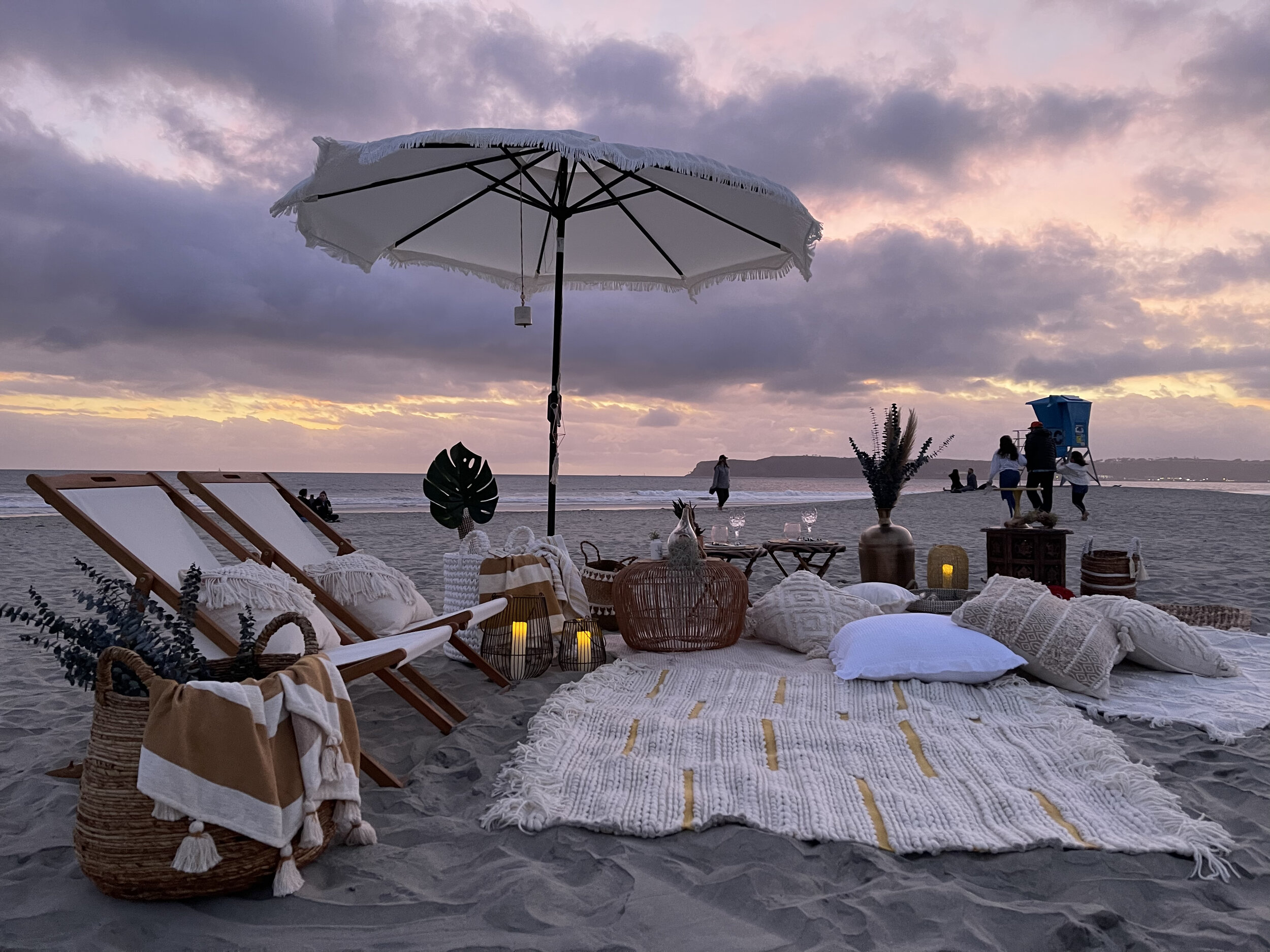A tranquil beach scene unfolds under a captivating twilight sky, tinged with hues of purple, yellow, and grey, suggesting an approaching storm or the transition into night. A prominent white umbrella fixed on a black pole stands at the center, flanked by two wooden beach chairs draped in white cloth with cushy white cushions. To the right, a white rug adorned with numerous pillows lies invitingly, while a wooden basket containing a brown-and-white towel and some foliage rests nearby. Scattered around the setup, two small tables each holding a wine glass hint at recent enjoyment. Although no people are seated in the immediate area, the overall arrangement — complete with a couple of packages, potted plants, and a standing beach towel — exudes a lived-in, comfortable vibe. The serene ocean with gentle waves stretches under the sky, with a faint mountain range visible in the background, and a blue structure and some people can be spotted on the right side. The beach, characterized by its clean, brown sand, also features a life guard chair, indicating an area of supervised relaxation or activity. Despite the absence of the beachgoers, the carefully arranged scene suggests they might be nearby, perhaps strolling along the shore or engaging in beachside activities.